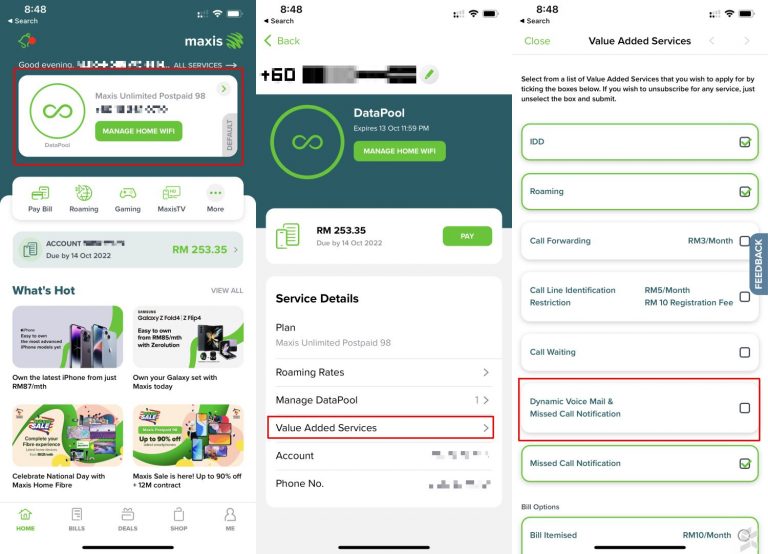**Image Description:**

The visual interface displays a comprehensive summary of a mobile service account, primarily for the telecom provider Maxis. Key features and indicators include:
- A partially filled signal strength indicator.
- Strong Wi-Fi connection and almost full battery life.
- The carrier name, Maxis, and a greeting message “Good evening, all services.” 
- The plan name “Maxis Unlimited Postpaid 98.”
- A red-bordered icon labeled PayPal, alongside icons for roaming, gaming, and Maxis TV.
- A gray oval showing an account due amount of MYR 253.35 by 14th October 2022.
- Promotional text encouraging celebration of National Day with Maxis Home Fiber and highlighting up to 9% off with an ongoing contract.
- A notification from sender "+60" indicating account details including a datapool expiry on 13th October at 11 pm.
- Options to manage the home Wi-Fi and view service details such as roaming rates and value-added services.
- A list of value-added services like IDD, roaming, call forwarding, call identification, call waiting, dynamic voicemail, missed call notification, and itemized billing.
- Instructions to select or unselect additional services as needed, by ticking the respective boxes.

Essentially, this image encapsulates a user-friendly dashboard summarizing account details, service plans, upcoming payments, promotional offers, and options for managing additional services.